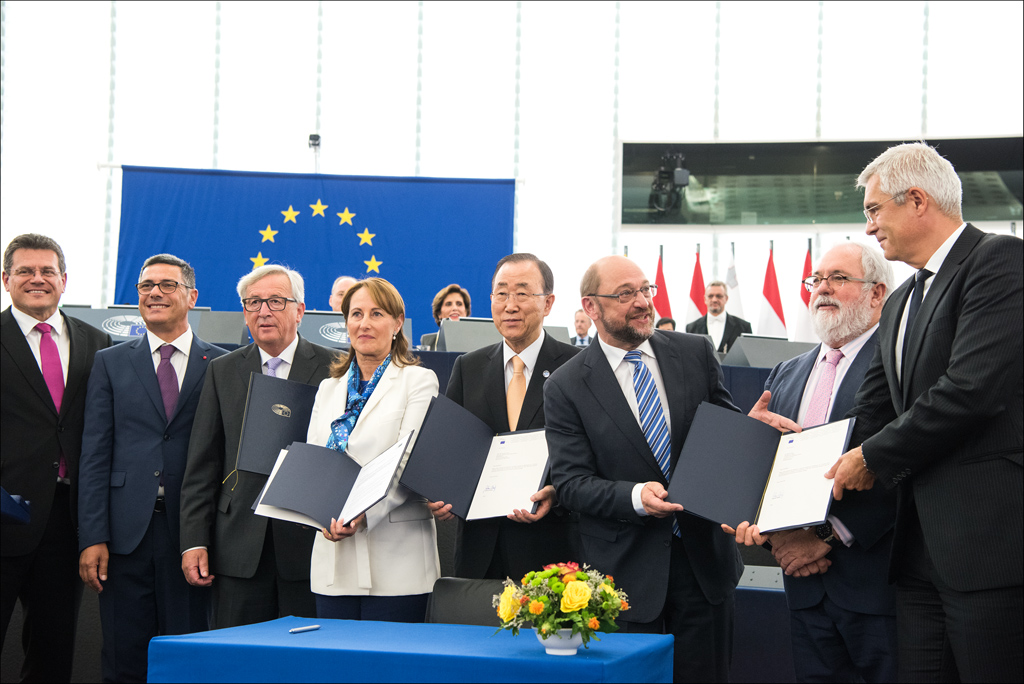This photograph captures a significant signing event, where eight prominent individuals are gathered at a blue-draped table adorned with a delicate arrangement of flowers and an elegant pen poised for action. The group in the foreground consists of seven men and one woman. The men are sharply dressed in a mix of black and navy suits with coordinating ties. The woman stands out in a sophisticated white jacket complemented by a vibrant blue scarf. Each person holds a navy folder containing pristine white documents, signaling the importance of the occasion.

In the background, the setting is further embellished with a series of red and silver flags and a prominent blue flag featuring gold stars, which adds a sense of formality and patriotic pride. The backdrop of the scene is a pristine white wall that frames a clear glass window, allowing for natural light to contribute to the excellent image quality. The photograph captures every detail with clarity, making it easy to distinguish the participants and their ceremonial roles in this important moment.